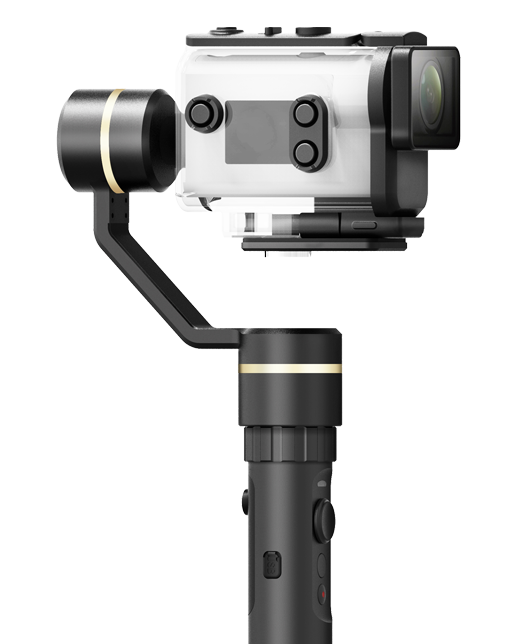The image displays a compact video camera mounted on a black gimbal, which functions similarly to a selfie stick but provides more stable movements. The gimbal starts with a straight vertical rod that curves diagonally to the left before extending upwards to connect with the camera via a golden or off-white ring. The gimbal features several buttons: three positioned on the lower part and possibly one at the back. The camera, predominantly silver with black accents around the lens and buttons, is affixed to the arm of the gimbal. The camera lens, housed within a square glass protective casing, is evident from the side angle view, which also reveals a secondary transparent square casing with three circular buttons on the side. The entire setup, which is centrally framed against a white background, includes an additional circular ring in a golden or off-white hue at the top of the gimbal.